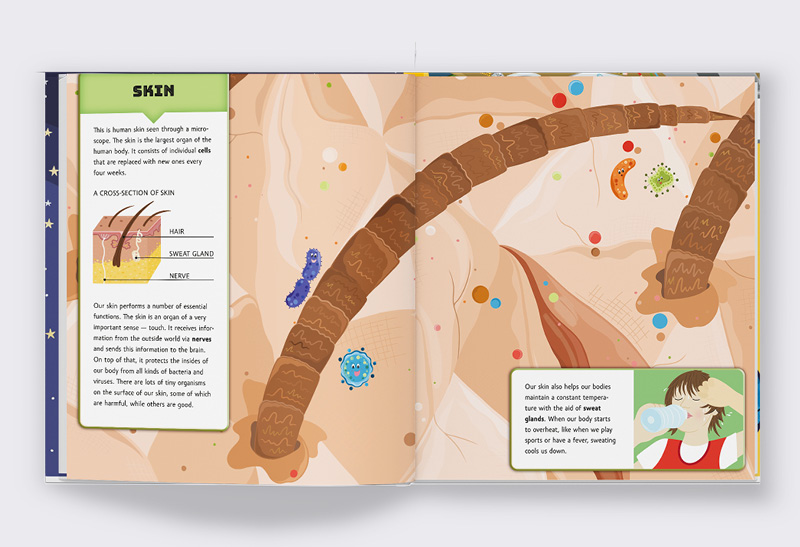The image depicts an open book, seemingly a children's educational book, showcasing an informative spread about human skin. The left-hand side of the pages contains textual information, explaining that human skin is the largest organ of the body, viewable through a microscope, and comprised of individual cells that regenerate every four weeks. The text emphasizes that skin helps maintain constant body temperature through the activity of sweat glands. On the right side, there's a large, detailed illustration spanning both pages; it features a magnified cross-section of skin, highlighting a single hair follicle. Surrounding the follicle are colorful, animated representations of bacteria and germs, drawn in a whimsical, child-like style with faces. The diagram labels various skin components, including nerves, hair follicles, and sweat glands. At the bottom right corner, an illustration of a person drinking water underscores the importance of staying hydrated to aid skin function. The page overall combines engaging visuals with educational content to teach readers about the structure and importance of skin.